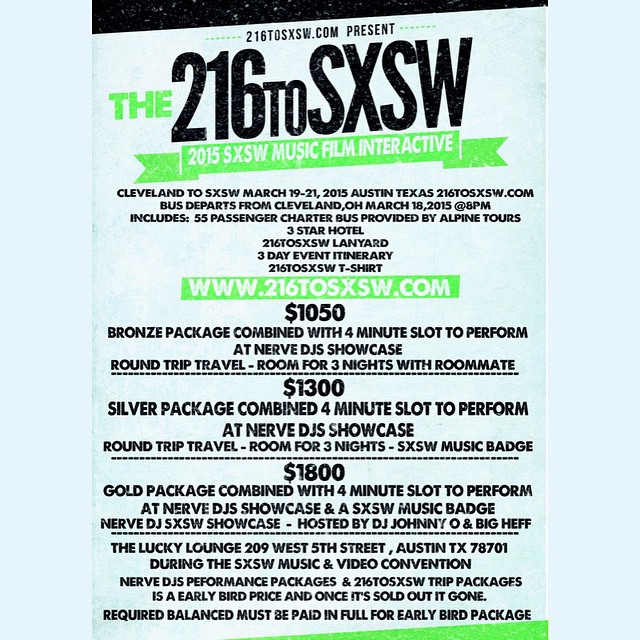This is a detailed paper advertisement poster primarily in white, featuring a black band at the top with some lime green accents. At the top, in large black letters, it says "216 to SXSW," and below it, "2015 SXSW Music Film Interactive." The poster is promoting a sponsored bus service from Cleveland to the South by Southwest (SXSW) festival in Austin, Texas, scheduled for March 19-21, 2015. The bus departs from Cleveland on March 18, 2015, at 8 p.m., provided by Alpine Tours in a 55-passenger charter bus, with accommodations at a 3-star hotel for three nights.

The poster offers three travel packages: 
1. **Bronze Package**: $1,050, includes a 4-minute performance slot at the NERV DJ Showcase, round-trip travel, and a shared room for three nights.
2. **Silver Package**: $1,300, includes a 4-minute performance slot at the NERV DJ Showcase, round-trip travel, a shared room for three nights, and an SXSW music badge.
3. **Gold Package**: $4,800, includes a 4-minute performance slot at the NERV DJ Showcase, a shared room for three nights, an SXSW music badge, and special mention at the NERV DJ SXSW Showcase hosted by DJ Johnny O and Big Hef. 

The events and performances will be held at The Lucky Lounge, located at 209 West 5th Street, Austin, TX 78701. Additional details and an address for more information are provided at the bottom of the poster.